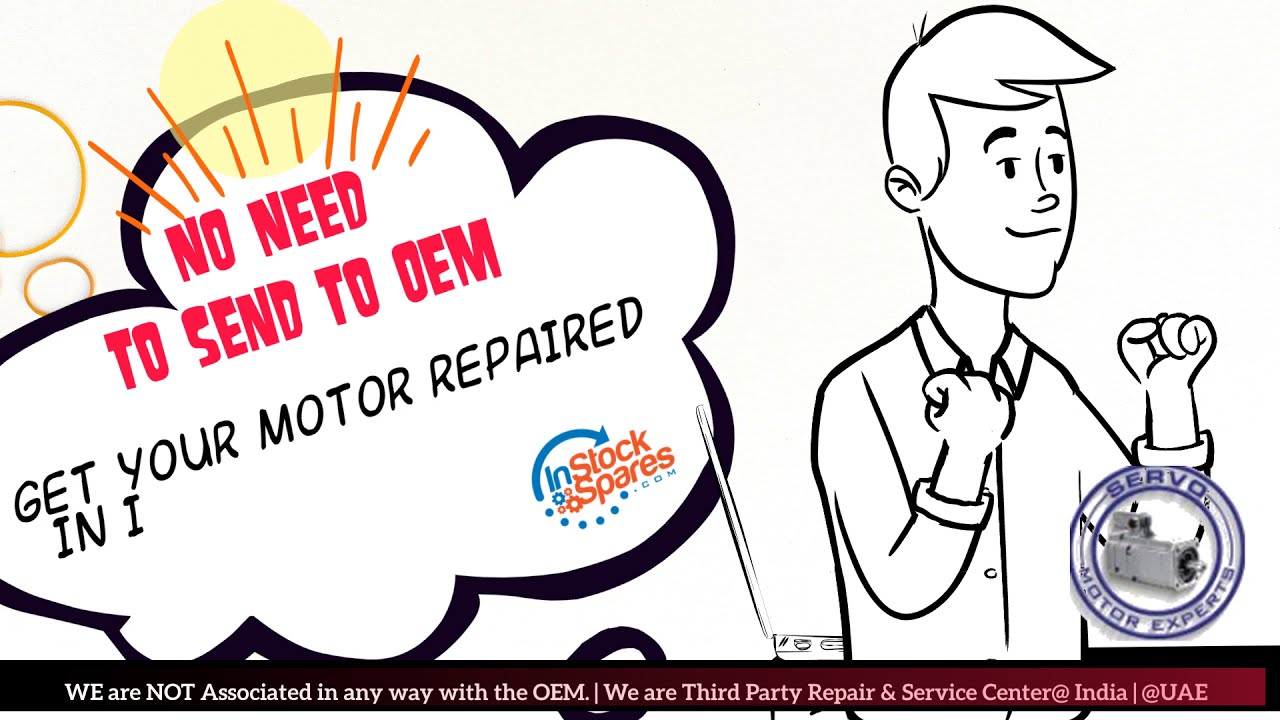The cartoon image features two main characters: a cloud on the left and a man on the right. The background is predominantly white with black linework, accented with touches of red, yellow, blue, and orange. The central figure, a man with short hair and a smirk, is depicted with raised arms and clenched fists, wearing a button-down long-sleeve shirt with the sleeves rolled up. To the left, the cloud contains reddish-pink text proclaiming, "No need to send to OEM," followed by black text stating, "Get your motor repaired in I," and a logo that reads "In Stock Spares" in blue and orange with an arrow motif. Below the logo, a banner transitions from black to red, declaring, "We are not associated in any way with the OEM. We are a third party repair and service center at India, at UAE." In the lower right corner, there is a blue logo featuring a piece of machinery and the words "Servo Motor Experts."